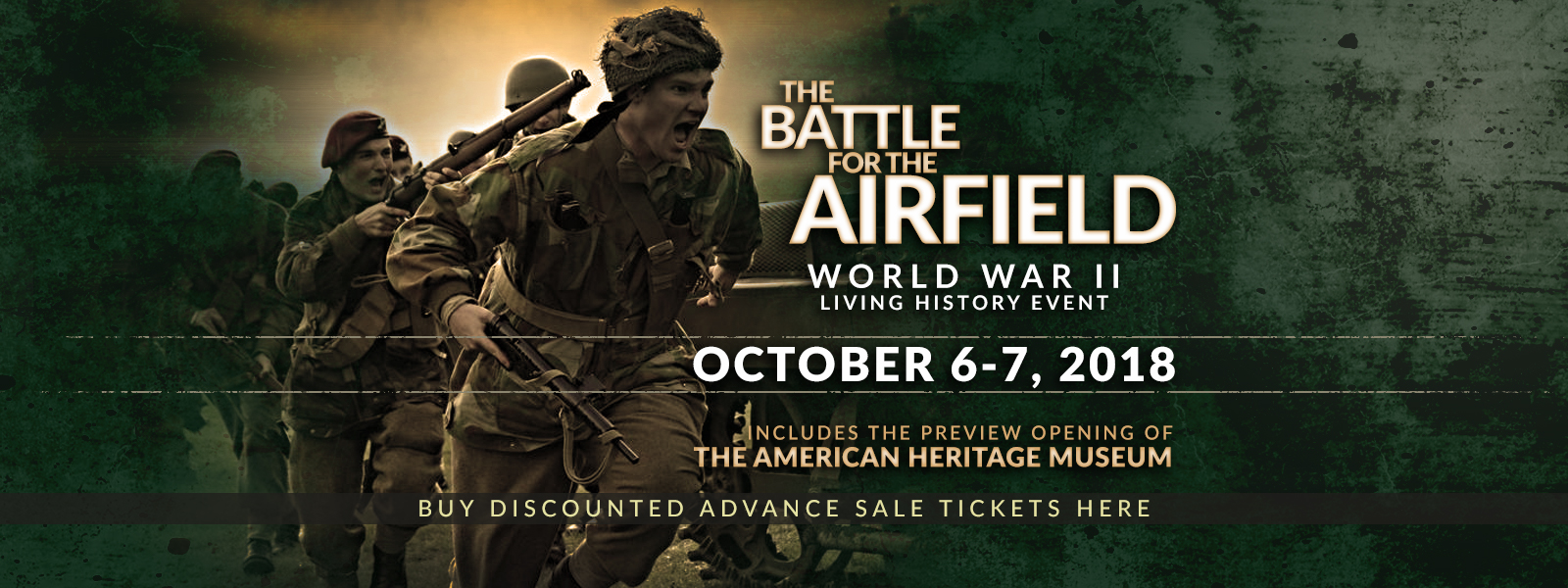The image is a promotional poster for the "Battle for the Airfield," a World War II living history event held on October 6th and 7th, 2018, which also features the preview opening of the American Heritage Museum. The poster's design prominently displays the event's title in white and yellow bold letters, with "The Battle for the Airfield" in white and "for the" highlighted in yellow. Below the title, the event dates are written in white between two yellow lines. Additional information, including "Includes the preview opening of the American Heritage Museum" and "Buy discounted advance sale tickets here," is written in yellow on a gray strip. The left side of the poster features an image of soldiers in camouflage uniforms, armed and running, evoking a sense of urgency and action. The right side of the poster shows green colors with some black stains, contributing to the overall wartime aesthetic.